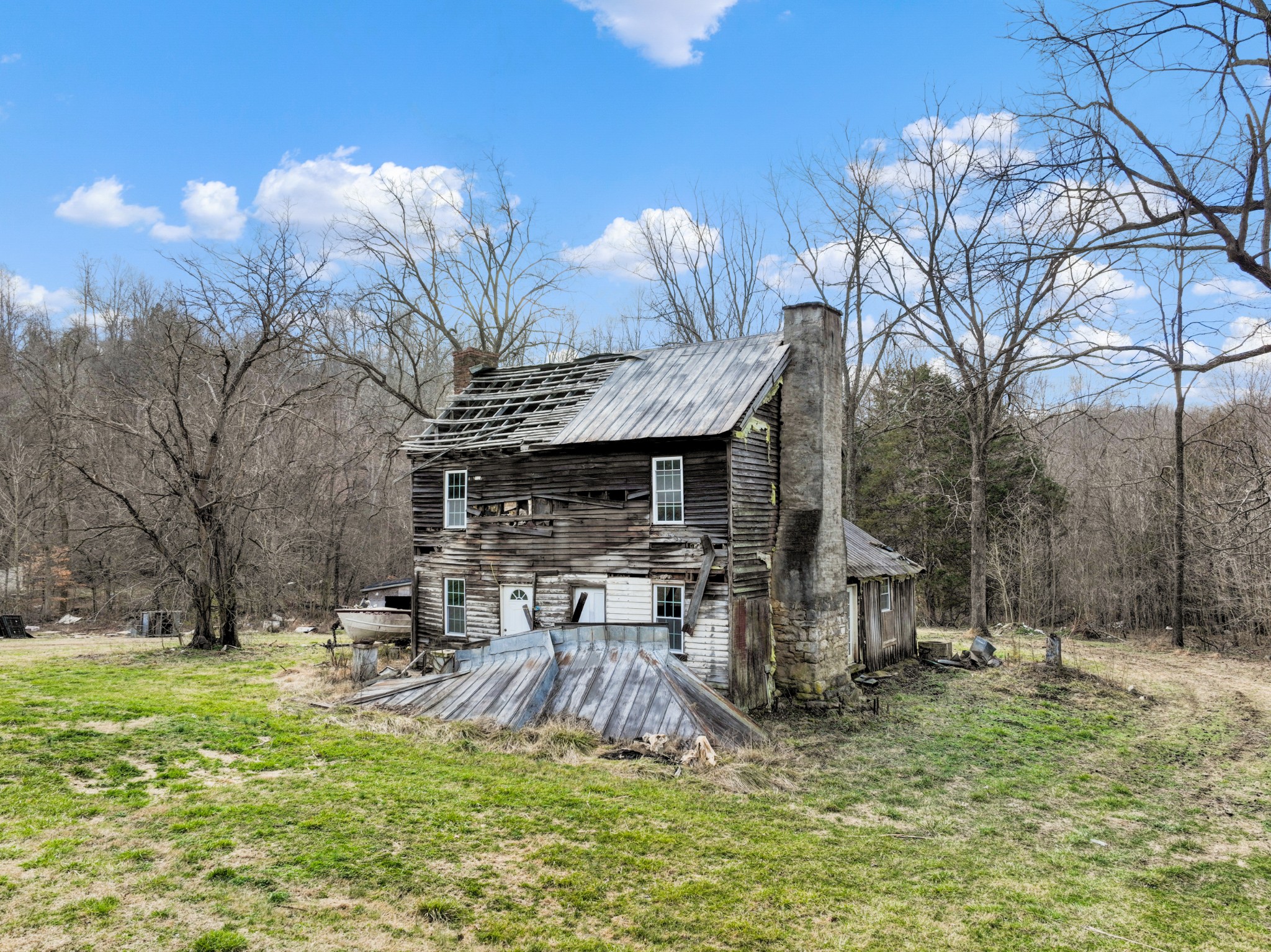The image depicts an old, dilapidated two-story house, likely located in a rural area. The house, which seems to have once been painted white, is now weathered to a predominantly wood-toned appearance with remnants of white paint at the base. The structure looks particularly precarious, with a significant portion of the roof missing on the left side, exposing the interior to the elements. 

On the right side, there remains a tin-covered section, but the overall state of disrepair suggests it's far from being protective. The wooden exterior is deteriorating, with planks falling apart and visible holes providing a glimpse into the abandoned interior. Two tall brick chimneys are notable, one on each side of the building, although their stability matches the fragile state of the rest of the house. 

In the foreground, a patchy, non-lawn green grass area extends towards what appears to be a trailing boat junked beside the house, adding to the scene's desolation. This sailboat on a trailer is positioned to the left, indicating neglect. Surrounding the clearing, a thick, leafless forest forms the backdrop, suggesting the season might be late fall or winter. This setting further enhances the forlorn and forgotten ambiance of what perhaps was once a quaint cabin.